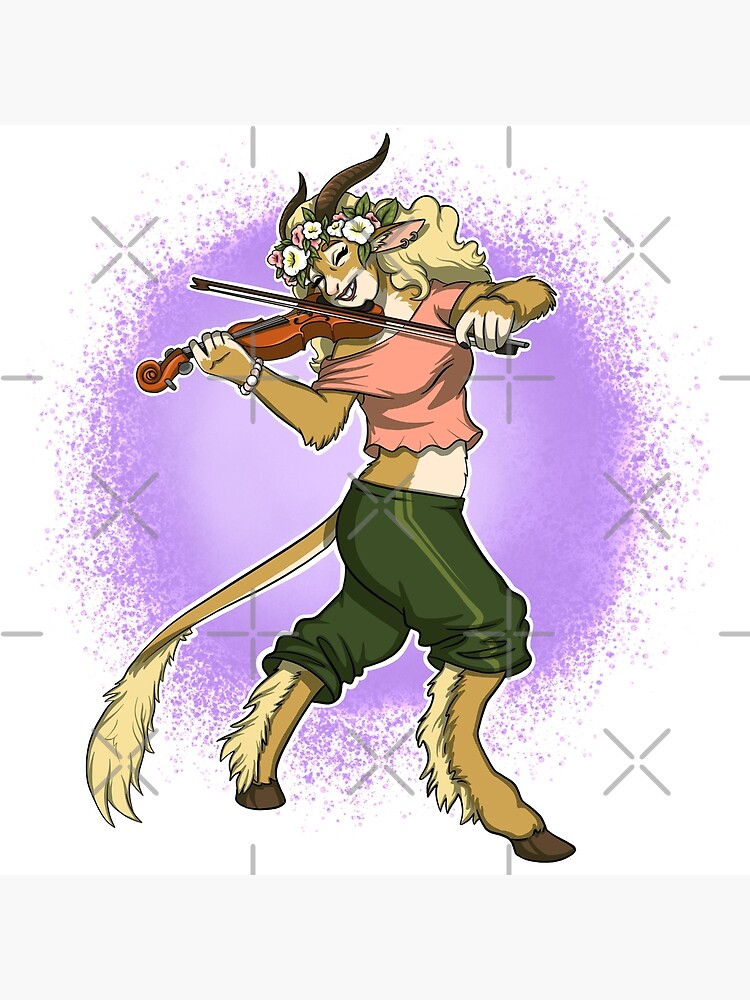The image is a colorful cartoon drawing of a female character that is a whimsical blend of human and animal features. She has the stance and legs of a horse, complete with hooves, and a long tail reminiscent of a lion's. Her arms and hands are human-like, while her face combines human and lion-like traits, adorned with long, sheep-like ears and black, curved antlers. She wears a wreath of white and pink flowers around her golden, flowing hair, adding a delicate touch to her wild persona. The character is joyfully playing the violin, a radiant smile on her face, and appears to be dancing. She is dressed in a light-colored, pink, off-the-shoulder top that reveals her midriff and green sweatpants that are pulled up to her knees. A white bracelet adorns her wrist, adding to her charming and playful appearance. The background is predominantly white, featuring a splattered purple circle that makes the character stand out vividly, highlighting her happy and carefree spirit.